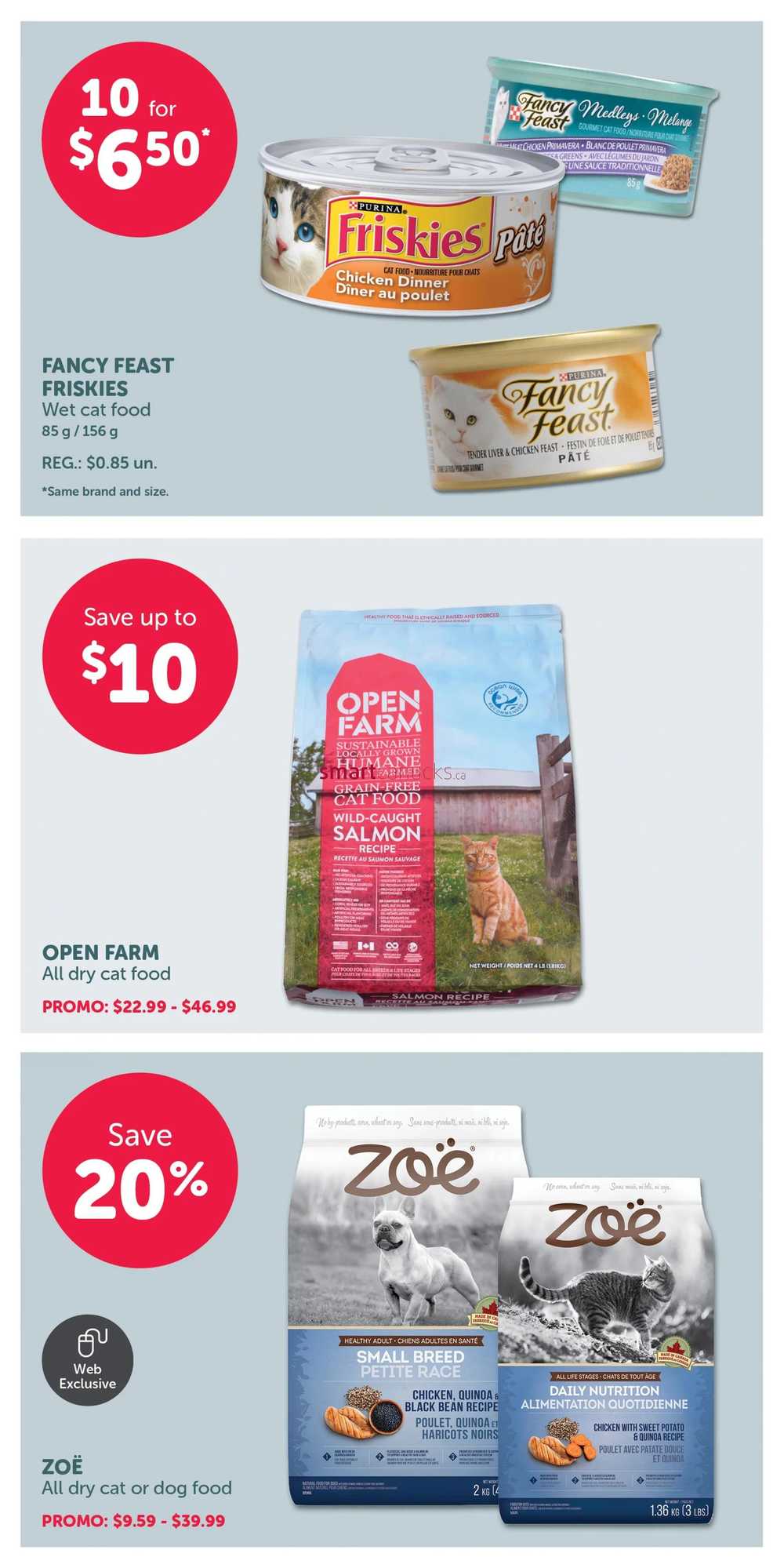The image consists of three vertically stacked pictures, each separated by a thin white border approximately a quarter of an inch.

1. The top image has a light grayish-blue background. In the top left corner, there is a red circle with bold text that reads "10," followed by smaller text saying "4" and "6 dollars for fifty-six or fifty cents." In the bottom right corner, black lettering states "Fancy Feast Friskies," along with "wet cat food," and the sizes "85G / 156G." The price indicates the same brand and sizes. To the right of this text, there are three cans of cat food displayed: the central can features a large "Friskies" label, while the cans to the top left and bottom right are labeled "Fancy Feast."

2. The middle image features a light gray background with a large red circle in the top left corner, containing the text "Save up to $10" in bold white letters. To the right, a big paper bag for cat food is depicted, showing an orange cat against a blue sky with green grass and a brown fence in the background. There's a red tab down the right side of the bag with white information. In the bottom left corner, it says "Open Farm" followed by "All dried cat food" and a promotional price range in red that reads "$22.99 to $46.99."

3. The bottom image has a slightly darker gray background. In the top right corner, a red circle with the text "Save 20%" is visible. There are two bags of pet food: the central bag, designed for dogs, has a gray top part and a blue bottom part, while the bag on the right is for cats. Both bags are branded "ZOE." Below the red circle, there is a black circle labeled "Web exclusive" in white text, with the green text "ZOE" underneath. Below that, "All dry cat food" and a promotional price range of "$9.59 to $39.99" are listed.